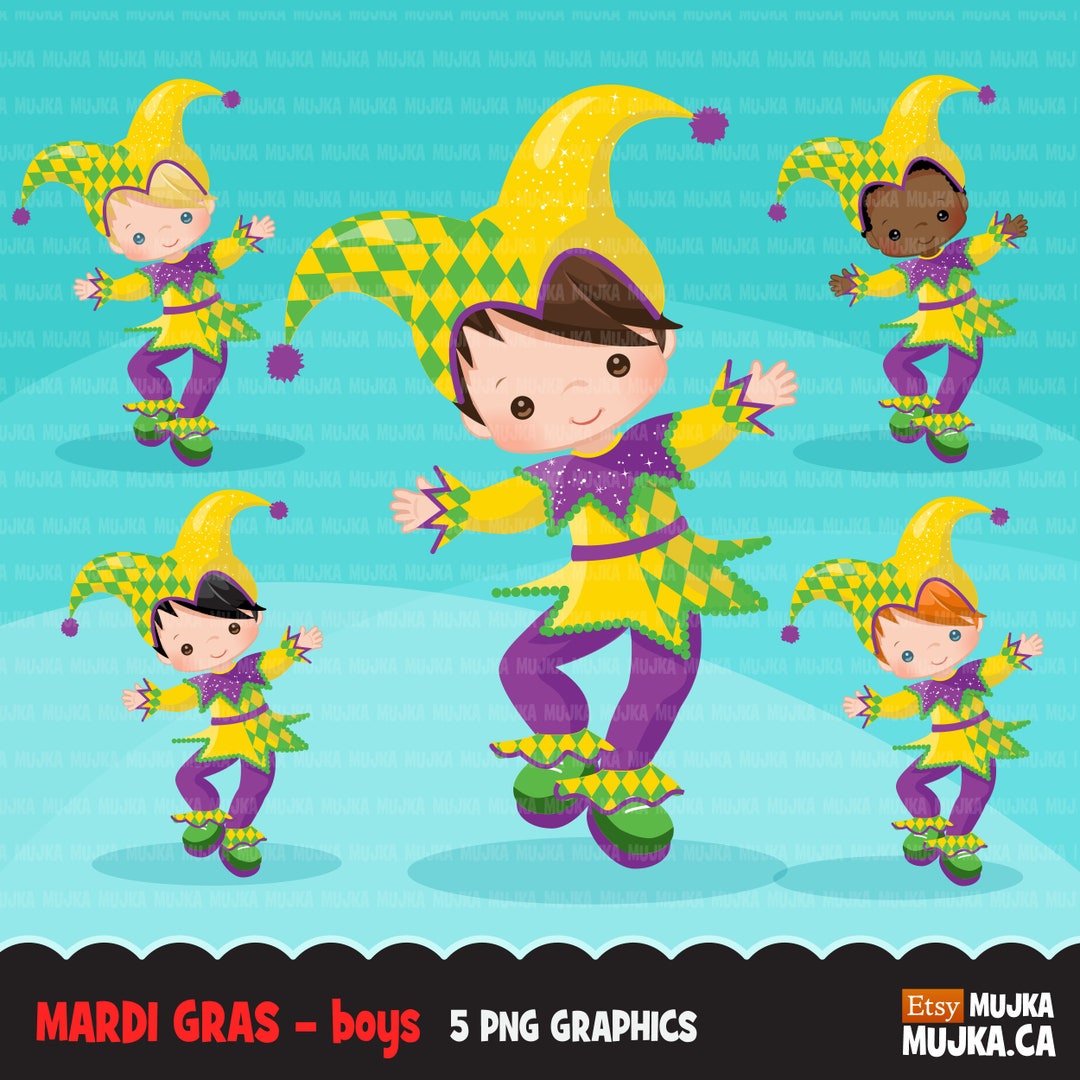The image features a light blue background with a faint, repeated watermark reading "moochka.ca" in tiny text, accompanied by the Etsy logo set against an orange square. At the center of the illustration is a cartoon child with brown hair, donned in a playful jester outfit, complete with a yellow and green checkered jester hat accented by two purple puffs at the ends. This central figure is depicted dancing alongside four other cartoon children, each unique with varying skin tones and hair colors: blonde-haired in the upper left, black-haired in the lower left, brown-skinned in the upper right, and light-skinned with red hair in the lower right. All characters are clad in similarly whimsical jester costumes, a quintessential blend of Mardi Gras colors—purple, green, and yellow. These characters, drawn with playful expressions and lively movements, give the impression they are celebrating exuberantly. Below the dancing figures, a black bar with a wavy border runs horizontally, featuring the text "Mardi Gras Boys" in bold red letters, followed by "5 PNG Graphics" in white, all in capital letters.